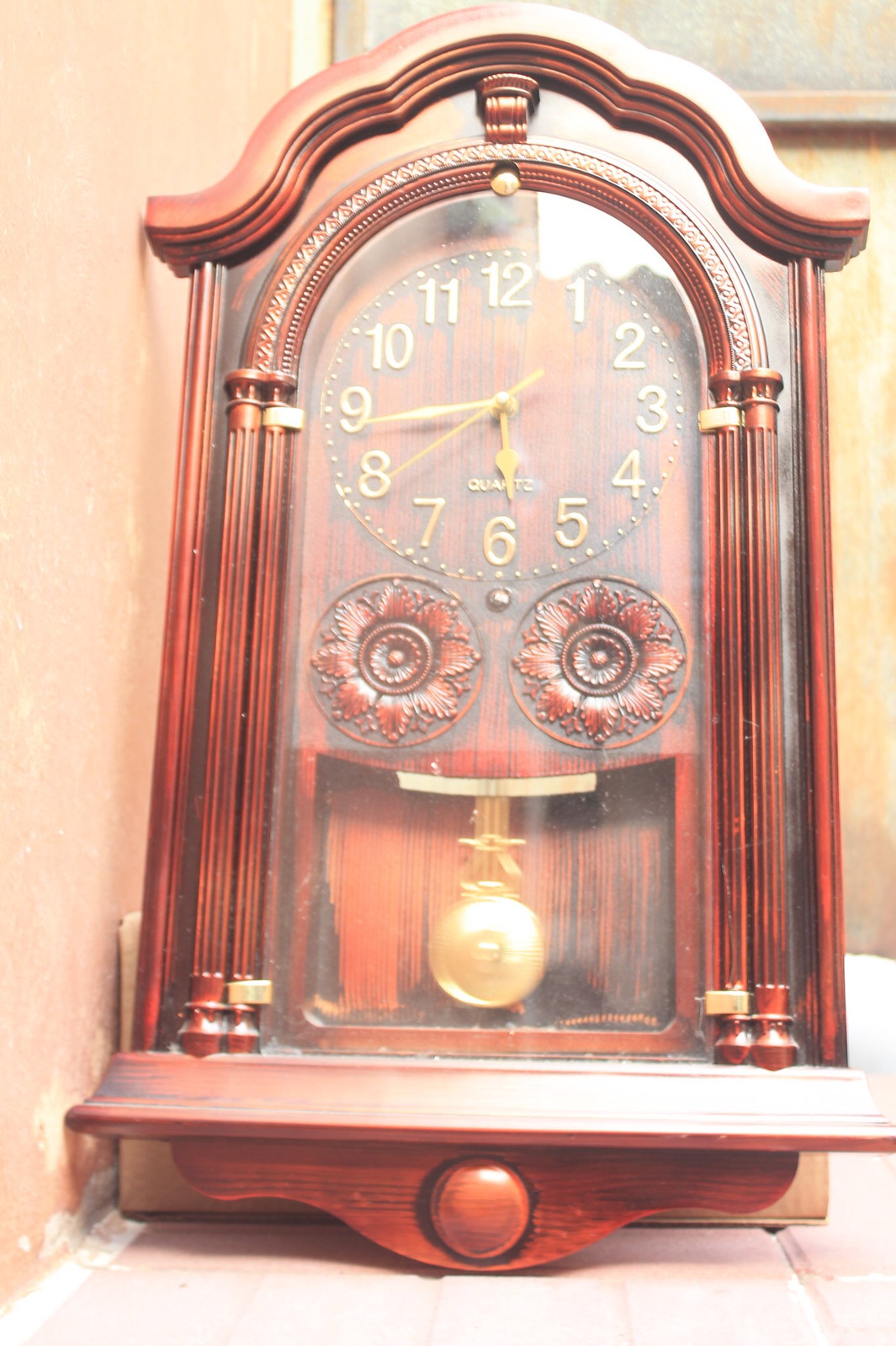The image showcases a meticulously crafted small wooden clock reminiscent of a grandfather clock. The clock's structure is fashioned from a bright, rich burgundy wood that boasts a highly polished and shiny surface. The clock's face, encased within a reflective glass cover, displays classic white numerals ranging from 1 to 12, complemented by yellow clock hands. Below the clock face, two floral-like designs, matching the clock's deep burgundy hue, add an elegant touch. Centrally located in the clock's midsection is a golden dial, further enhancing the clock's sophisticated aesthetic.